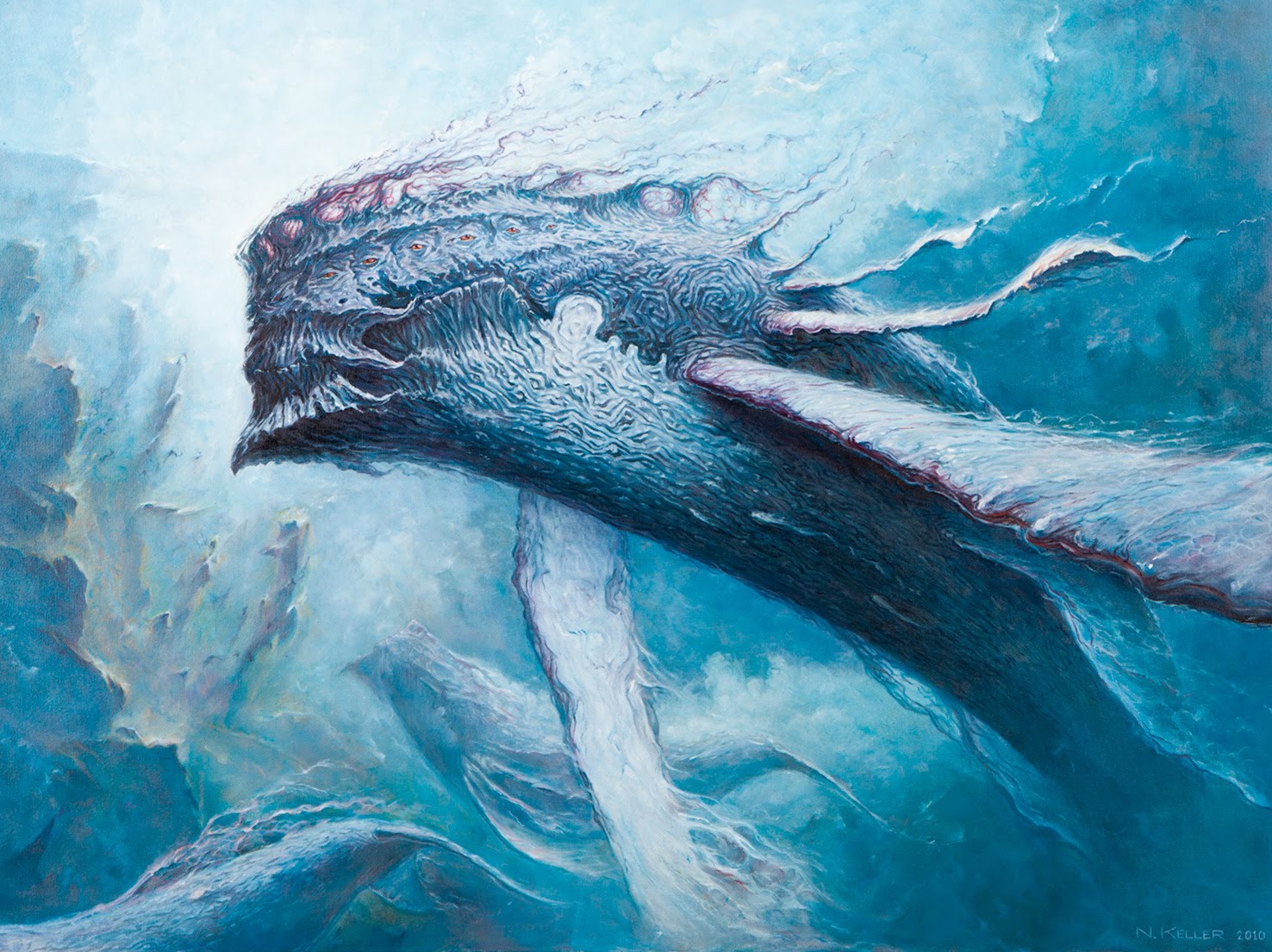This digital painting depicts three alien-like, whale-inspired underwater creatures against a light, almost cloud-like blue background that suggests a submerged world. The scene is rectangular, with the longer sides at the top and bottom. The main creature, positioned prominently in the center foreground, is covered in round ridges and sports an enormous fin on either side, which is twice as long as its body. Above these large fins are two smaller ones. The creature's large face, adorned with multiple red eyes and tendrils sprouting from the top of its head, contrasts with its blending blue body that melds seamlessly into the watery backdrop. This face ends flatly, without the typical whale's features, adding to its alien mystique. The background showcases a gradient with a lighter shade of blue in the top left corner merging into a darker hue in the bottom right, creating an effect of sunlight filtering through the water. Distantly, two other similar creatures float, adding depth and a sense of scale to the scene. Additional touches of pink blend with the blue and white highlights, giving the entire image a surreal, otherworldly feel.